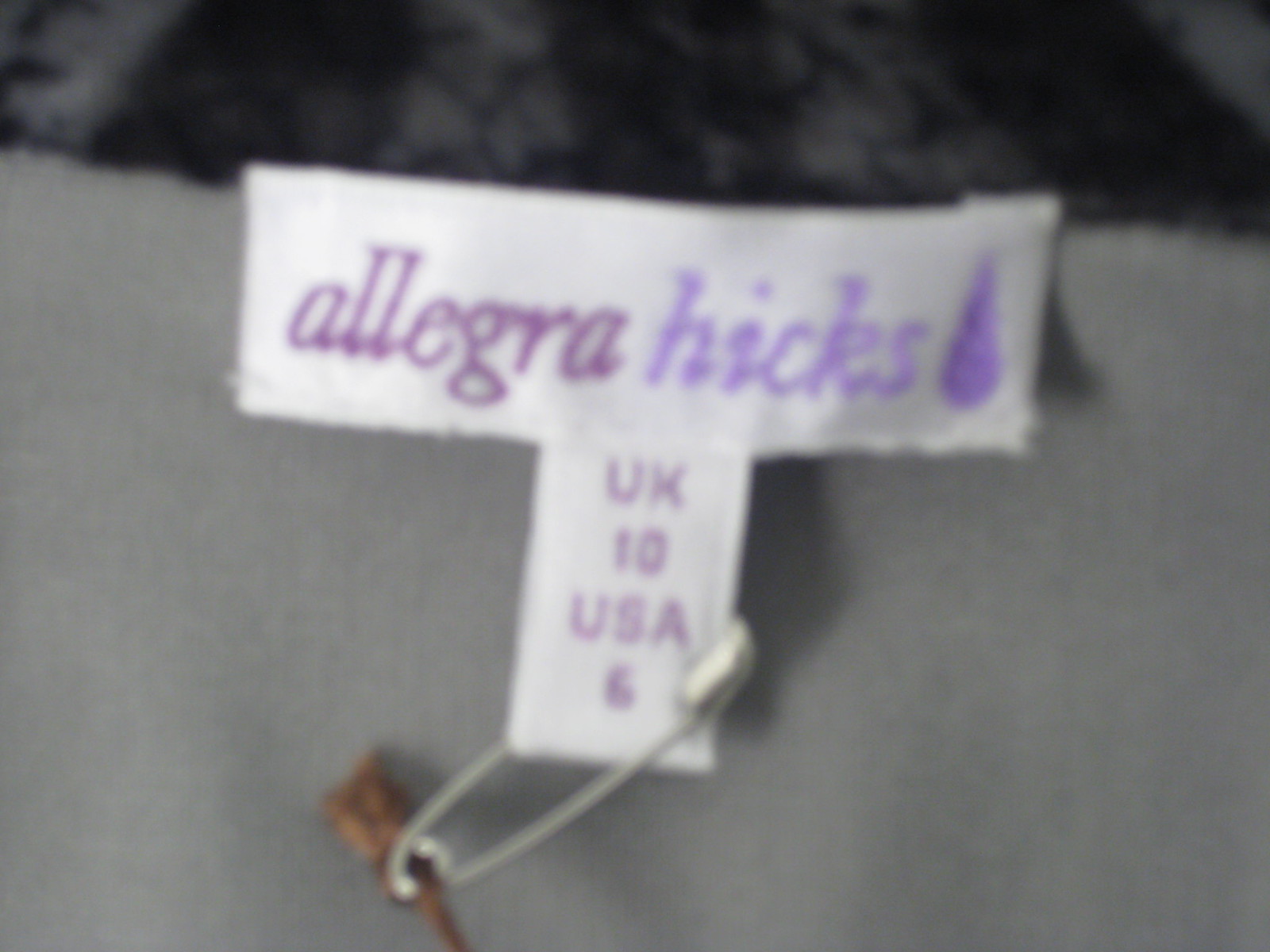This image showcases a blurry photograph of a clothing label attached to a gray fabric item. The label itself is white and rectangular, prominently displaying the brand name "Curse of Allegra" in darker purple, alongside "Hicks" in a lighter purple font. To the right of the brand name, there is an eyedrop-shaped symbol in light purple. Below this, a size tag hangs, indicating the sizes UK10 and USA6 in dark purple text against a white background. A safety pin is visible, securing the bottom of the size tag, with a brown object threaded through the pin. The upper part of the photo is mostly black and blurry, providing little contextual detail about the background.